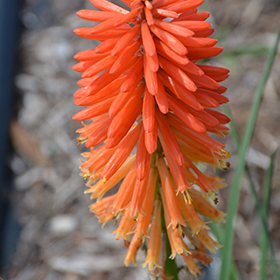This close-up image focuses on a cluster of narrow, tubular petals or structures of a flower, which exhibit a gradient from bright orange at the top to a more yellowish hue towards the bottom. The petals extend from a central point, radiating outward in various directions—downward, horizontally, and slightly diagonal—eventually exiting the frame both at the top and bottom. The background is extremely blurred, offering a hint of a natural scene with diffuse green stalks, likely grass, on the right, and a mix of indistinct whitish-tan elements suggestive of foliage or branches. Despite the lack of any written labels or objects for scale, the detailed close-up brings an intense focus to the fine structure and vibrant coloration of the flower's petals.